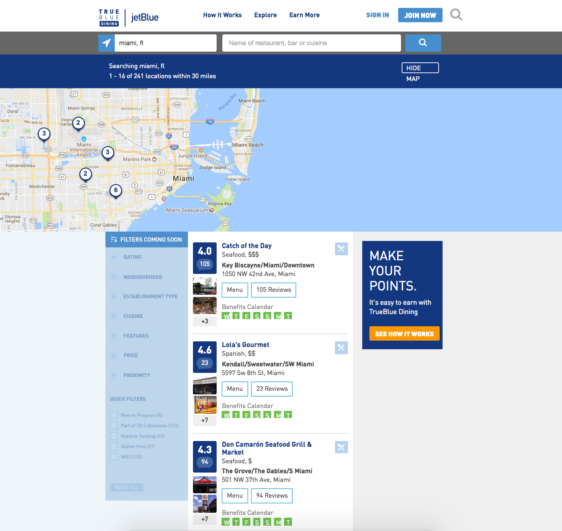This is a detailed caption for the provided image:

"A screenshot of the JetBlue website page showcasing its interface. At the top, the website features the JetBlue logo in bold blue letters on a white background, followed by a navigation bar with various tabs. One of the clearer tabs reads 'Explore More,' and next to it, another tab labeled 'Even More.' The remaining tabs are somewhat blurry and difficult to decipher.

Below the navigation bar, there appears to be a search bar designed for users to look up specific flights or destinations. This is followed by a prominent map with a blue background. The map itself is depicted in shades of gray, interspersed with orange lines and white circles featuring dark blue indicators. Additional splashes of green and light blue add more detail to the map.

Right underneath the map, the screen is divided into three sections. On the left side, there is a long, blue rectangle that is very blurry and illegible. Next to it on the right, another long rectangle, which is almost double the width of the first, contains noticeable content. This section features ratings for different restaurants: a 4.0 rating for 'Catch of the Day,' a 4.6 rating for 'Lala's Gourmet,' and a 4.3 rating for an establishment named 'Southern Grill and Marketplace.' Each restaurant name is followed by its respective rating, providing a clear overview of dining options."